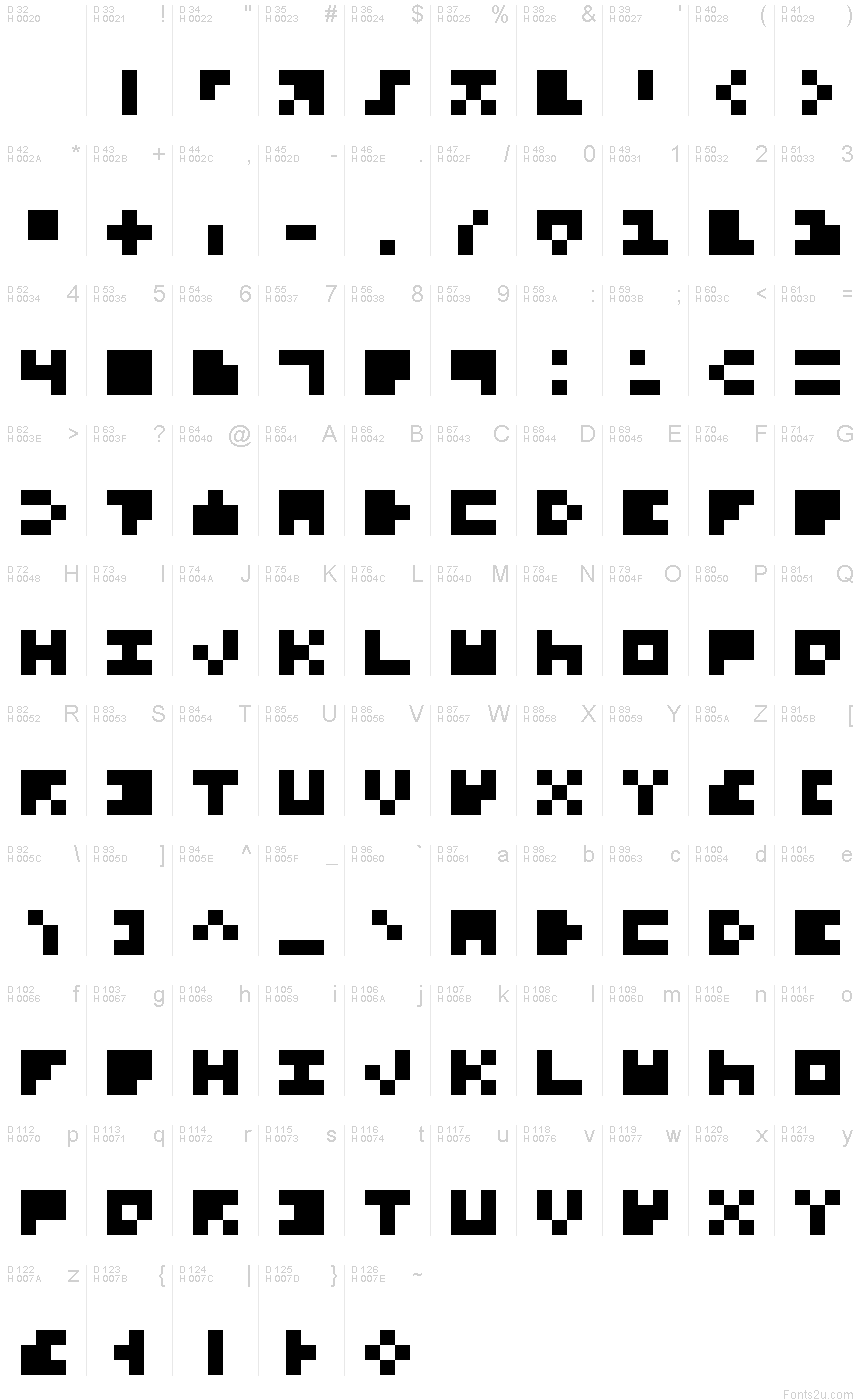In this particular image, we see a screenshot of a computer desktop displaying a grid composed of 10 columns and 10 rows. Each column appears to contain 10 characters, except for column 1 which contains 9 symbols, and similarly, each row has 10 characters except row 1 which also contains 9 symbols.

The grid consists of various symbols including squares and lines through squares, each of which is marked by an alphabetized system ranging from A to Z, followed by four additional characters that are numbered differently. Some of the characters also feature numerical Japanese writing, adding a layer of complexity and detail to the symbols displayed. The overall appearance is that of an intricate arrangement of symbols on a computer screen, carefully organized and distinct in its presentation.